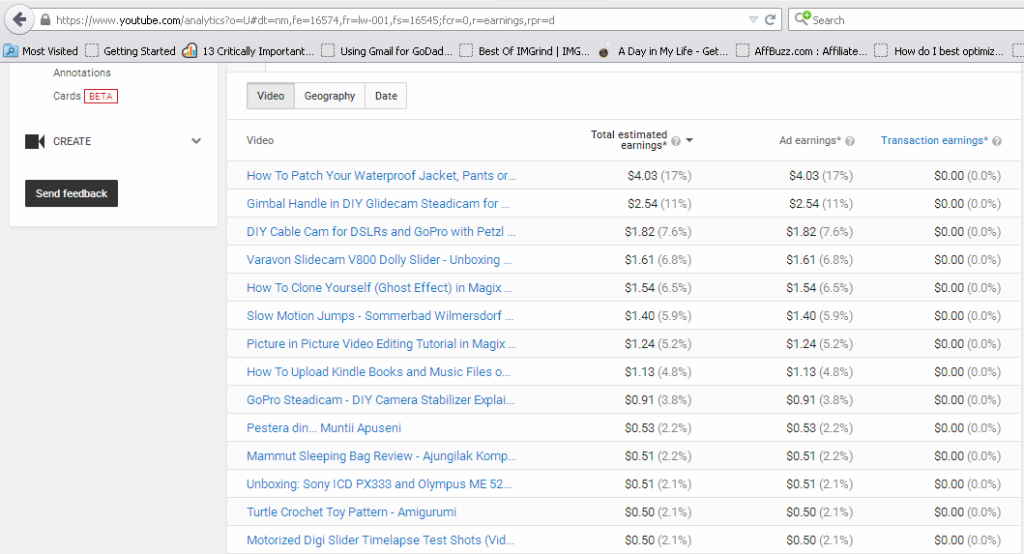Here is a detailed and cleaned-up caption for the image:

"The image displays a comprehensive breakdown of YouTube.com analytics, highlighting the most visited sections. Key topics include 'Getting Started,' '13 Critically Important Tips,' utilizing 'Gmail for GoDaddy,' and top content from 'mgrind' and 'mge.' Additional entries feature 'A Day in My Life,' 'fbuzz.com Affiliate Strategies,' and optimization techniques for annotations, cards, and beta features. Tutorials cover a range of subjects such as patching a waterproof jacket, handling gimbals, and constructing DIY equipment like glide cams, steady cams, and cable cams compatible with DSLRs and GoPros using Petzl Vaviron. There are also guides on building slide cams, dolly sliders, and achieving effects like cloning, ghosting, and slow-motion jumps. Other highlights include a review of the summer in Wilmersdorf, video editing tips incorporating picture-in-picture and various effects, as well as instructions for uploading Kindle books and music files to GoPro. The list extends to DIY camera stabilizers, explanations on past events, a review on compact sleeping bags, and unboxing videos for Sony ISD PX333 and Olympus ME52. Product tests for motorized digisliders and timelapse techniques are also covered, with detailed technical specifications including: AS 403 2.54, 1.82, 1.61, 1.54, 1.41, and intricate decimal figures for performance measurements."